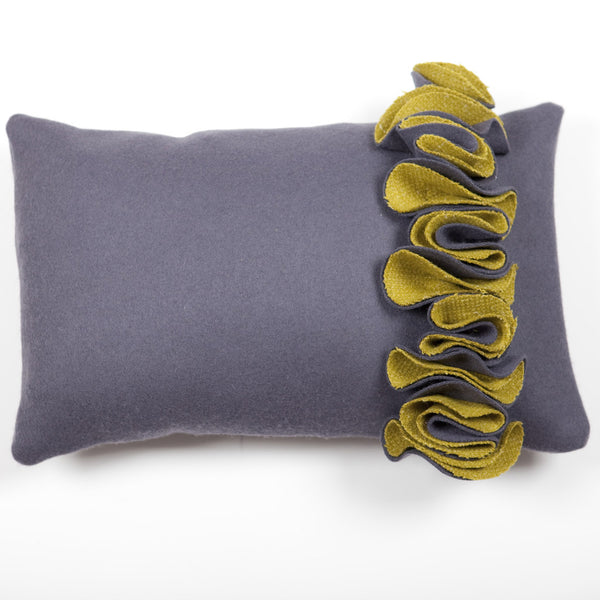This is a detailed photograph of a rectangular, grey pillow positioned centrally against a solid white background. The pillow features four pointed corners and casts a subtle shadow on the surface beneath it, suggesting a soft standard fabric without a separate cover. The most distinctive element of the pillow is an intricate decorative frill located on the right side. This embellishment consists of grey fabric, matching the pillow's primary color, and reveals hints of green within the ruffles. The frill is artfully arranged, resembling scrunched-up fabric that evokes the appearance of overlapping flower petals or interconnected "U" shapes. This unique, stitched-on decoration adds visual interest and a touch of elegance, aligning with bedding or fabric design aesthetics.